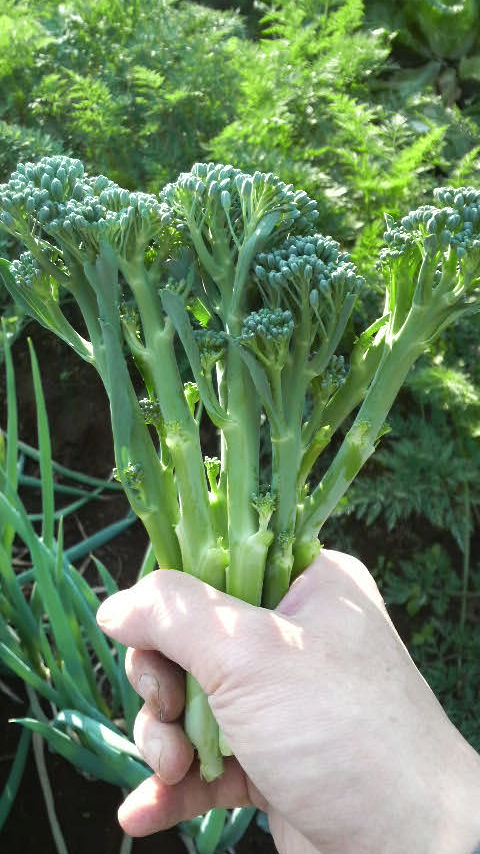In this bright, sunny, outdoor scene, a Caucasian hand, slightly weathered and gripping freshly picked broccolini—or broccaccini—is prominently featured. The broccolini, a long-stalked green vegetable often served as a side dish, appears freshly cut, with its dark green florets contrasting against the slightly lighter green stalks. The hand comes from the lower right corner of the vertically-oriented, rectangular photograph, indicating the person has been actively harvesting. The hand and nails bear slight dirt, suggesting work in the garden. In the background, bushes, trees, and long grass bathed in sunlight further evoke a sense of a warm, vibrant afternoon spent tending to the garden. The sun casts subtle shadows of the broccoli onto the hand, enhancing the vividness and detail of the image.